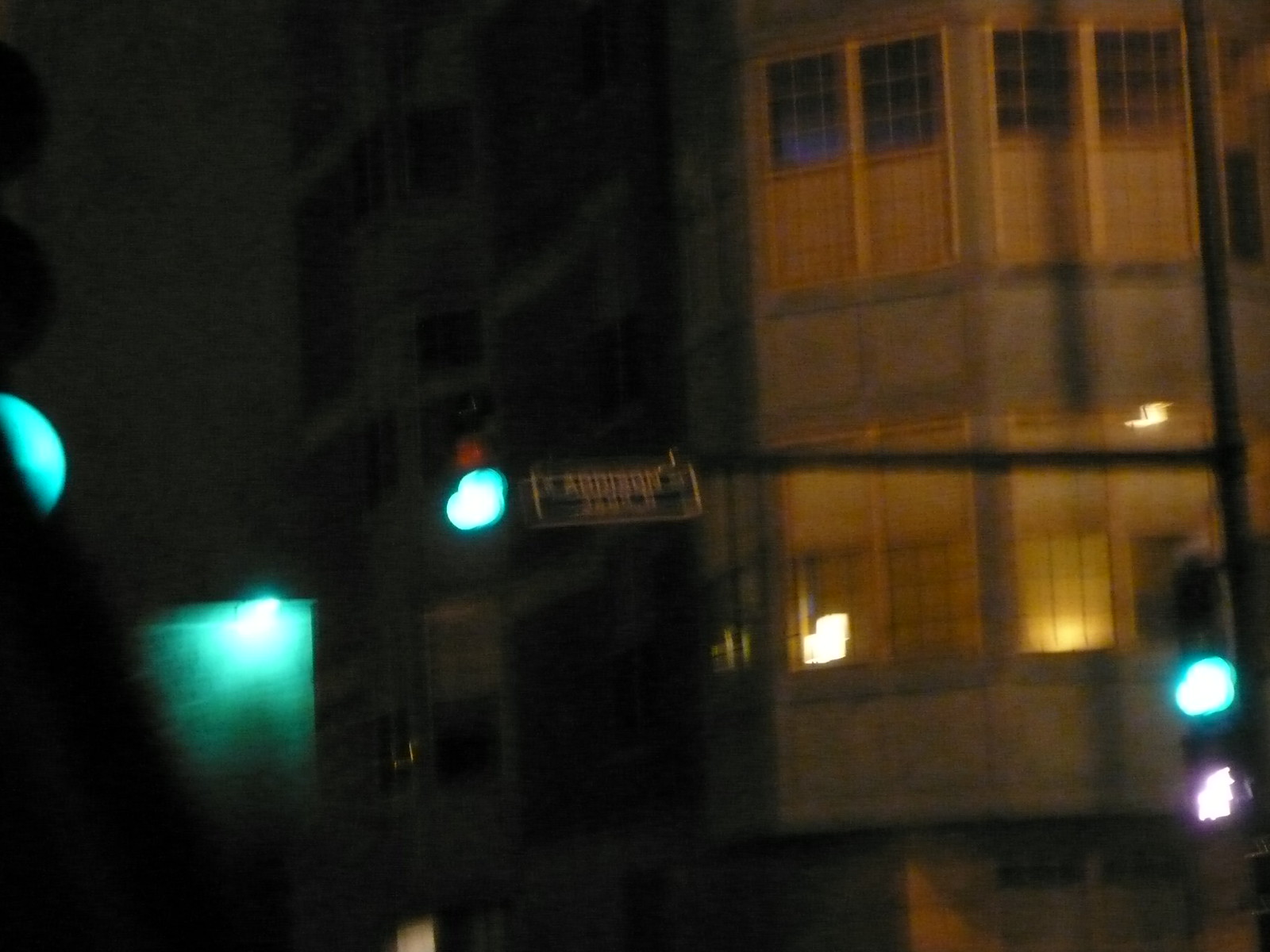A nighttime photograph with a distinct, grainy, and aged artistic feel. The most prominent feature is a green stoplight, suspended from a pole. Adjacent to the stoplight, there is a green and white metal sign. The backdrop is dominated by a colossal, light-colored building featuring several windows, some of which have lights on, illuminating the otherwise dark and quiet night. To the left, a portion of the same building appears, noticeably darker with none of its windows lit. A green light casts a reflection on a nearby surface, adding a subtle, eerie glow to the scene. Underneath the green stoplight, on the left side of the image, an illuminated sign is partially visible, casting a faint, mysterious light.